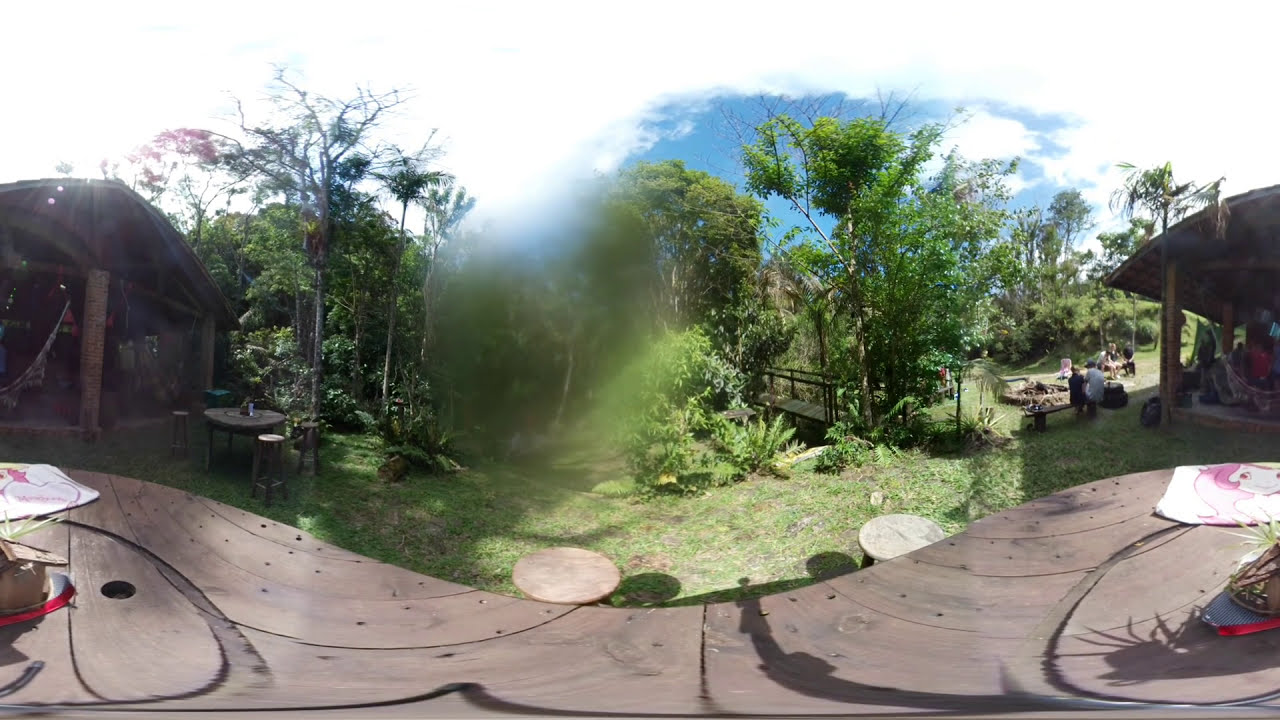The image portrays a picturesque outdoor picnic area captured with a wide-angle lens, causing some distortion and a noticeable blur or water droplet in the center. The scene is set under a partly cloudy sky with patches of blue and white clouds. The area features lush green lawns and a variety of tall, leafy trees that form a scenic backdrop. 

In the foreground, there's a grayish wooden deck adorned with picnic tables and wooden benches. One prominent table is draped with a white tablecloth, surrounded by four matching wooden chairs, also covered with white cloth. On the right side of the image, there's a circular fire pit and people engaged in conversation, likely sitting near a gazebo. The left side features a partly indoor, partly outdoor platform with more picnic tables and benches, where figures can be faintly seen. 

Beyond the wooden deck and to the right, there's a vertical wooden fence with small houses visible in the distance, and to the left, a similar fence flanked by vibrant greenery. A small leafy tree with a brown trunk is noticeable among taller, dense trees. Additionally, you can see a wooden bridge extending into the woods, adding to the idyllic charm of the setting. Scattered ferns and a blanket laid out on the deck further evoke a relaxed, inviting atmosphere.